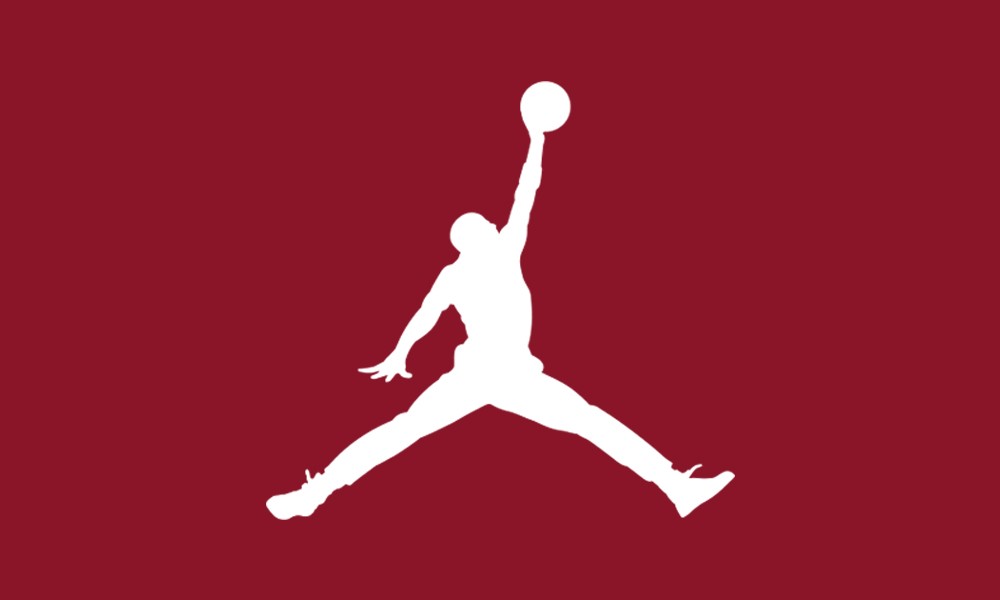The image features a horizontally aligned rectangle with a predominantly reddish to maroon background, centered perfectly with a striking white silhouette. This silhouette embodies the iconic image of Michael Jordan performing his legendary dunk. Jordan's legs are widely spread, his left hand raised high holding a basketball, and his right hand pointing downward with fingers splayed. Notable details include his prominently visible shoelaces and the distinctive pose that suggests the dynamic motion of leaping. The background lacks any textual branding like the Nike name or swoosh, implying this could be a self-made tribute by an ardent fan who admires both Nike and Jordan. The figure appears to be in full-length attire, possibly pants, adding a unique street-style aesthetic to the portrayal.